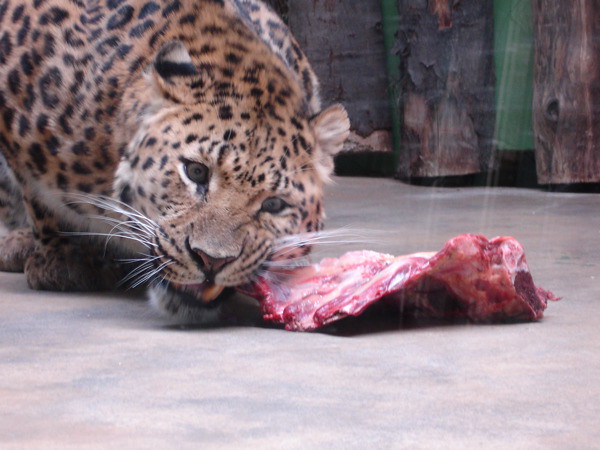The photograph captures a leopard crouched on a smooth gray and pink cement floor, partially facing the camera with a piece of red, marbled meat in its mouth. The leopard, an impressively large wild cat, showcases its striking orange fur adorned with several black spots, and an underside of white. Long white whiskers extend from its snout, which is in a slight snarl as it chews on rib bones within the meat. The backdrop features a log wall made of various carved, smooth logs, adding a touch of rustic texture to the scene. The image, likely taken in a zoo, offers a detailed view of the leopard's head, shoulders, and part of its body as it feeds.